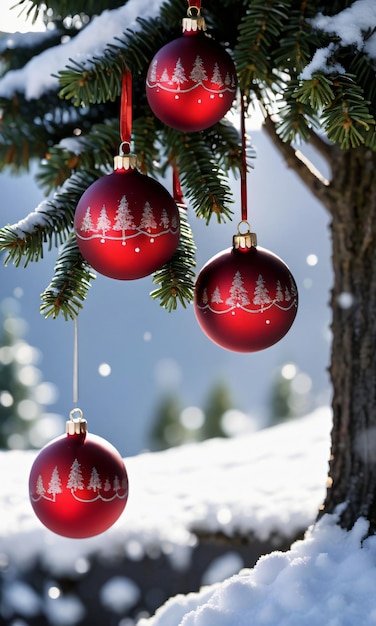This photograph captures a picturesque winter scene featuring four identical red Christmas bulbs adorned with white Christmas tree designs, hanging at various heights on an evergreen tree outside. The bulbs are secured with red ribbons to the snow-dusted branches of the tree, which is half-visible and reveals its rough, textured brown bark. Fluffy snow blankets the base of the tree, adding to the festive ambiance. In the blurred background, one can discern the outlines of distant green evergreen trees atop a snowy hill, set against a purplish-blue sky. Scattered throughout the image are subtle light blue or white circular highlights, adding a magical touch that enhances the wintry charm.